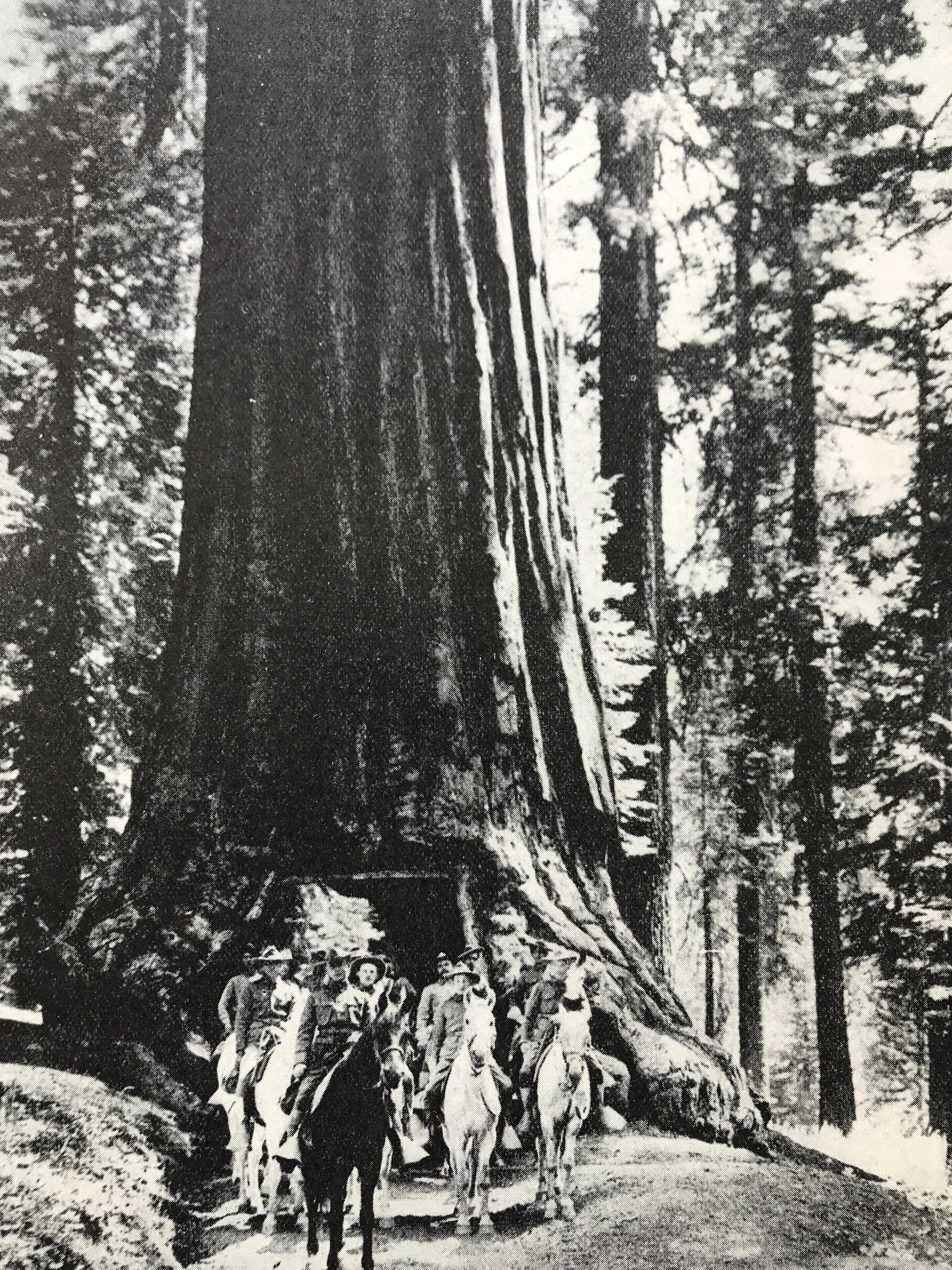The black and white photograph depicts an imposing scene, likely from a national park or a well-known location, featuring an enormous redwood tree with a hollowed-out center large enough for people to pass through. The focal point of the image is the tree trunk, with its carved-out passage that allows a group of uniformed individuals on horseback to navigate through. These individuals, dressed in attire reminiscent of Canadian Mounties or early 20th-century uniforms, ride beneath the canopy of leaves and branches that partially shade the area but still allow ample light to filter through. The riders, predominantly male, don wide-rimmed hats similar to cowboy hats. Leading the group is a rider on a black horse, with the others on white or off-white horses, traveling along a dirt path. The background of the photo includes scattered trees with moderate foliage, suggesting an open yet forested environment under a bright sky. The entire scene offers a historic glimpse into the majestic natural setting combined with a glimpse of human activity, possibly dating back around a hundred years.